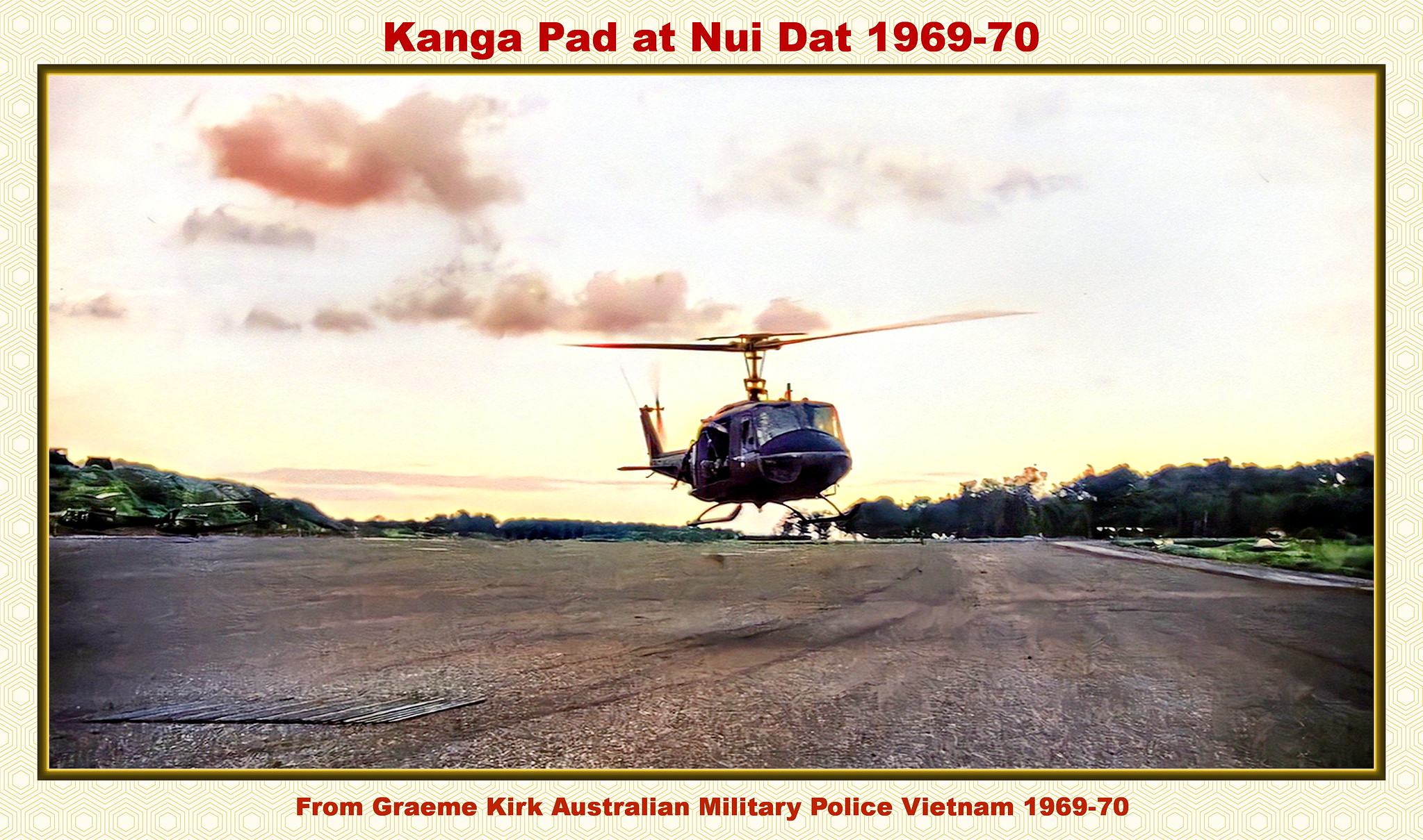The image resembles a postcard with a detailed and nostalgic layout. At the top, bold red text reads "Kanga Pad at Nui Dat, 1969-70," while at the bottom, similarly styled text states, "from Graham Kirk, Australian Military Police, Vietnam, 1969-70." The backdrop consists of a light yellow gradient adorned with white polka dots arranged within concentric hexagons. The central focus of the image is a helicopter, its rotors in motion, either landing or taking off on an expansive, paved area or runway. This scene takes place during what appears to be either sunrise or sunset, filling the sky with hues of yellow, gray, and orange and scatterings of clouds. To the left, distant vehicles or other helicopters are faintly visible, framed by patches of grassy terrain and trees. The setting provides a vivid glimpse into a moment from the Vietnam War, captured through a vintage lens, reflecting the distinctive environment and time period.